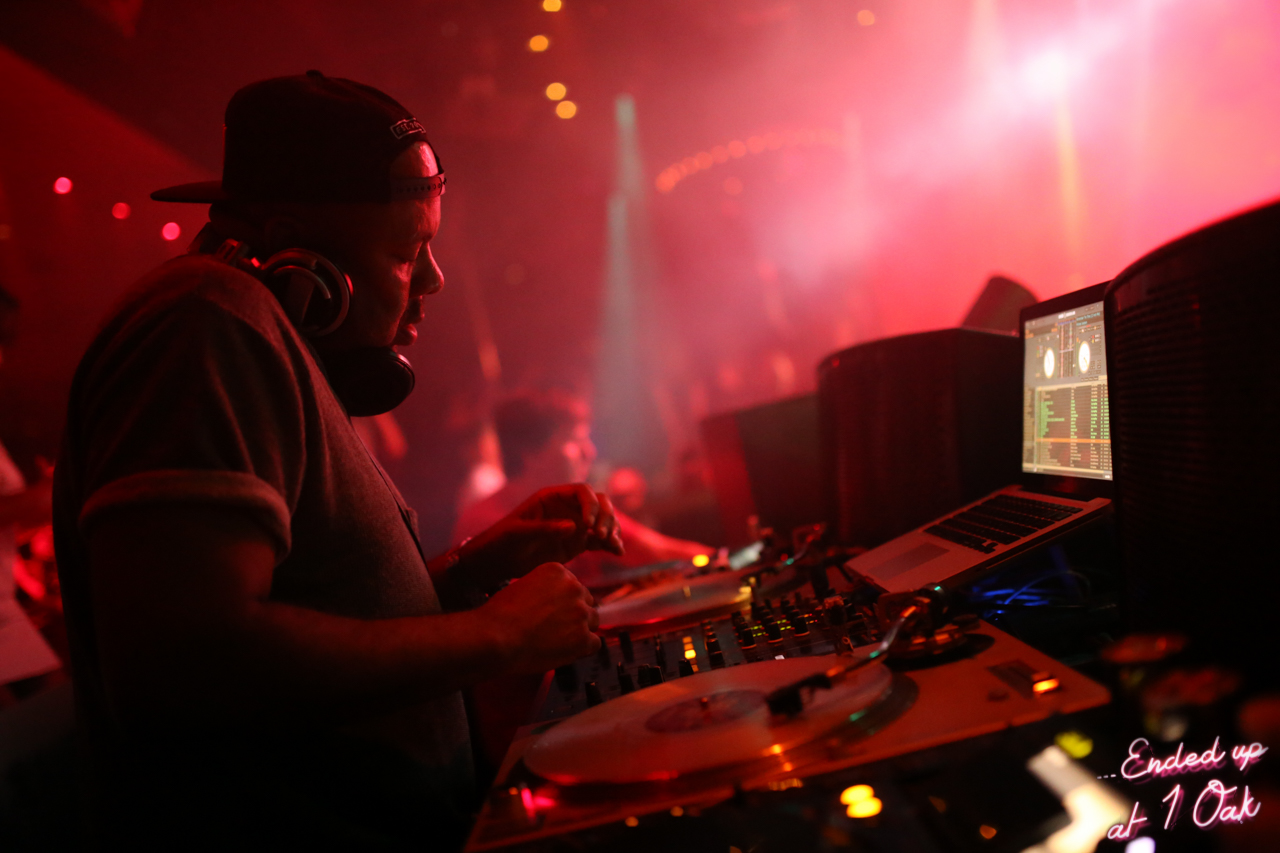In a dark, shadowy club scene illuminated by a mix of pink, red, yellow, and white lights, a DJ is stationed behind an array of electronic equipment. He wears a backwards black baseball cap and a t-shirt with rolled-up sleeves. His headphones rest on his head as he leans over his turntable and an open laptop, which displays various colorful graphics including white circles, green text, and an orange bar. The silver screen of the laptop stands out against the dark surroundings. To his left, a small pink light cascades down, and cursive text with a pink background in the bottom right corner declares, "Ended up at One Oak." In the background, silhouettes of people and additional light beams create a dynamic, lively party atmosphere.